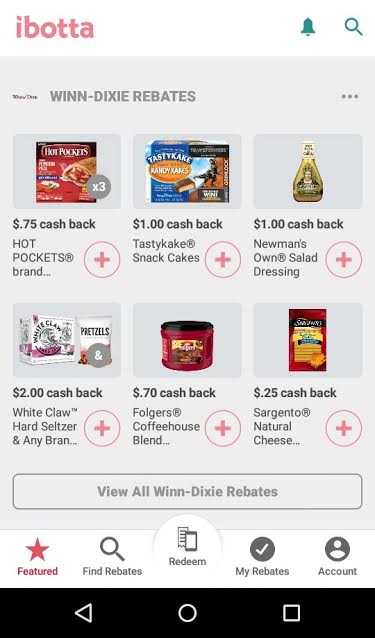This descriptive caption showcases the interface of a cell phone displaying the Ibotta application. 

---

**Detailed Caption:**

The image is a screenshot taken from an Android cell phone, evident from the wide black navigation bar at the bottom of the screen. This bar features three iconic Android buttons: a left-facing triangle for 'Back' on the left, a circle for 'Home' in the center, and a square for 'Recent Apps' on the right. 

At the top of the image, set against a white background, the app name "Ibotta" (I-B-O-T-T-A) is prominently displayed in the top left corner. Adjacent to this, on the right, there are two icons—a bell for notifications and a magnifying glass for search.

Occupying the majority of the screen against a light grey background are "Winn-Dixie Rebates," accompanied by the Winn-Dixie logo on the left. On the right, three vertical dots suggest additional options. 

Beneath this section are two rows, each featuring three product thumbnails. Each thumbnail includes a product image, a brief cashback detail, and a red circle with a plus sign, indicating the option to add the deal to the user's account. 

- The first row includes:
  - 75 cents cashback on Hot Pockets, marked with "times three."
  - $1 cashback on Tastykake Snack Cakes.
  - $1 cashback on Newman's Own Salad Dressing.

- The second row includes:
  - $2 cashback on White Claw Hard Seltzer.
  - 70 cents cashback on Folgers Coffeehouse Blend.
  - 25 cents cashback on Sargento Natural Cheese.

Below these rows is a grey block labeled "View all Winn-Dixie Rebates." 

Further down, a white strip presents additional navigation options. Starting from the left, the options include:
- "Featured," marked with a pink-lit star, indicating the current screen.
- "Find Rebates," denoted by a magnifying glass.
- "Redeem," represented by an image of a cell phone in the center.
- "My Returns," accompanied by a circle and arrow icon.
- "Account," symbolized by a circle with a line drawing of a person.

This image effectively showcases the Ibotta app's user interface, focusing on available rebates and the navigation options for users.